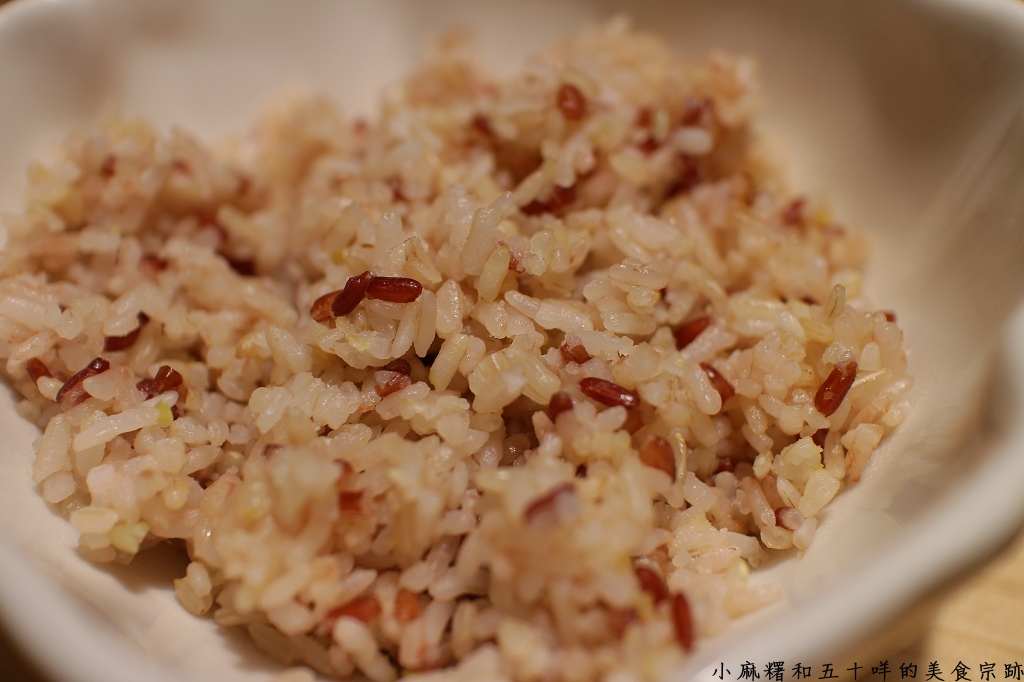This is a close-up, rectangular color photograph of a bowl of rice. The white ceramic bowl is set on a light wood-colored table. The rice itself is predominantly white, mixed with brown and reddish-brown grains, resembling a wild rice or pilaf dish. Small green flecks, possibly finely diced green onions, and tiny red flecks of seasoning are scattered throughout the rice, giving it a colorful and slightly textured appearance. In the bottom right corner of the image, overlaid black Chinese or Asian text can be seen. The close-up nature of the photograph leaves the background, including any potential utensils, out of focus and blurry.